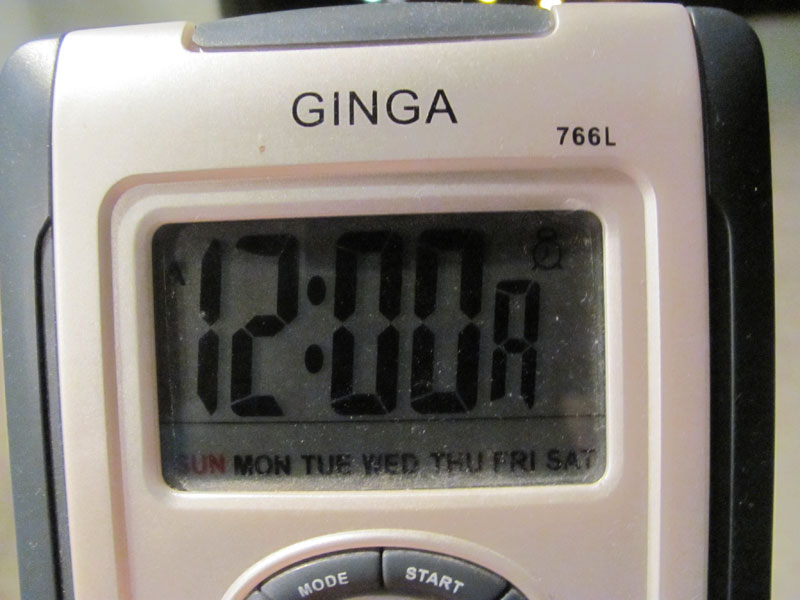In the image, a watch is prominently displayed against a solid gray background. The watch itself features a sleek design with varying shades of gray—ranging from light gray to darker tones. The brand name "Jenga" is clearly printed in black letters on the watch face. Additionally, the face displays the model number "766L."

The watch has a rectangular digital display window, which shows the time as "12:00 a.m." in clear black lettering. Across the bottom of the display, the days of the week—Sunday, Monday, Tuesday, Wednesday, Thursday, Friday, and Saturday—are listed sequentially. To the side of the display, a round dial is visible, flanked by light gray buttons. These buttons bear white text labels reading "Mode" and "Start," providing functional navigation controls for the digital watch.